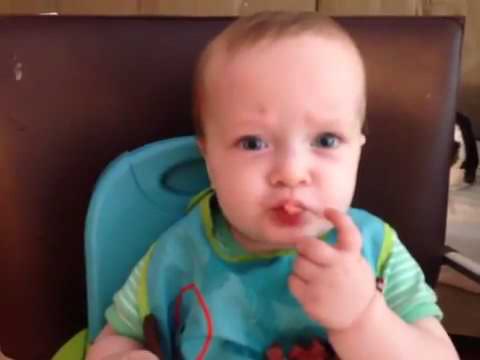This is a highly detailed photograph of a young Caucasian boy, approximately one to two years old, captured in an indoor setting. The focal point of the image is a close-up shot of the baby, centrally positioned, sitting in a light-blue, plastic high chair. The child, with big cheeks and puckered lips, is eating a small piece of food, possibly cereal, held delicately in his mouth. He sports a blue bib adorned with green accents over a blue and green striped t-shirt. His left hand is raised near his mouth, suggesting he might be pointing at or holding the food, while his right arm rests on the tray of the high chair. The baby has a light complexion, light blonde or brown hair, a large forehead, and light-colored, likely blue, eyes, which gaze directly at the camera with an expression of curiosity. The background features a dark brown wooden panel covering most of the space, and there appears to be a hint of a white table with an iron on it in the lower right corner, adding context and depth to the setting.